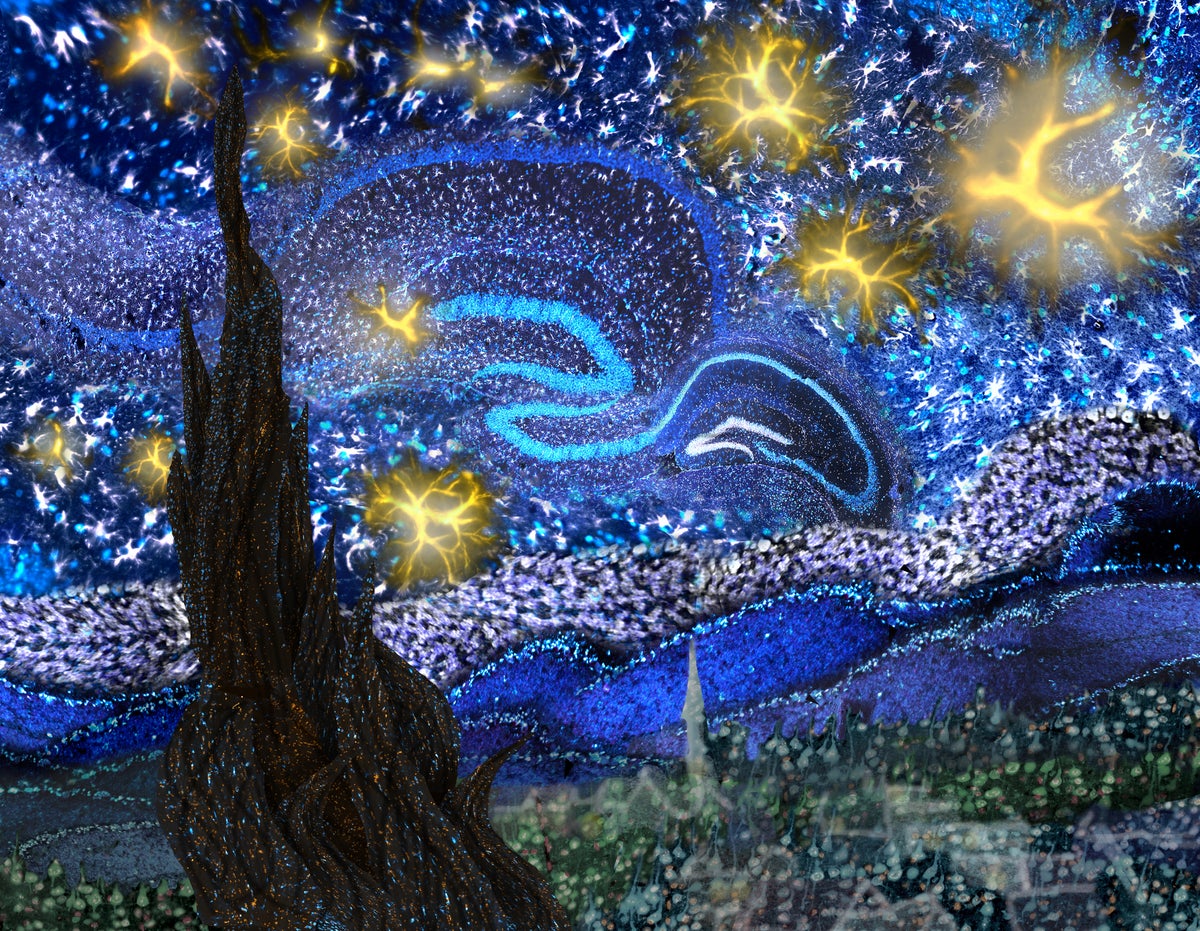This detailed painting, a modern reinterpretation of Vincent van Gogh's Starry Night with a touch of Pablo Picasso’s abstract influence, bursts with vibrant colors and dynamic patterns. The top portion shines with bright blue and white squiggly lines, interspersed with clusters of seven yellow lightning bolts that add an electrifying intensity, while four more bolts decorate the lower section. Dominating the right side is a brown, tree-like structure that resembles a branch of wood, adorned with reflective blue spots, evoking the enigmatic cypress from Starry Night. Surrounding the brown structure, various shades of green dots create a lively, textured backdrop.

Above this, dark blue waves interlaced with white undulate across the canvas, transitioning to a lighter blue sky speckled with white stars, lending a celestial ambiance. A pale section dotted with black specks introduces an intriguing contrast. On the left, there appears to be an abstract representation of a building structure ascending with the cityscape suggested by green, blue, and gray stipple marks below, conveying a night sky effect filled with vivid hues of light blue, dark blue, and even hints of purple. This composite painting creates a night sky teeming with life, invoking neural or fractal imagery, with yellow blobs that resemble neurons or brain cells, diffusing a sense of abstract thought intertwined with the cosmos. Overall, this piece is a luminous blend of Van Gogh’s iconic swirling patterns and Picasso’s abstract style, radiating with yellows, blues, and greens.